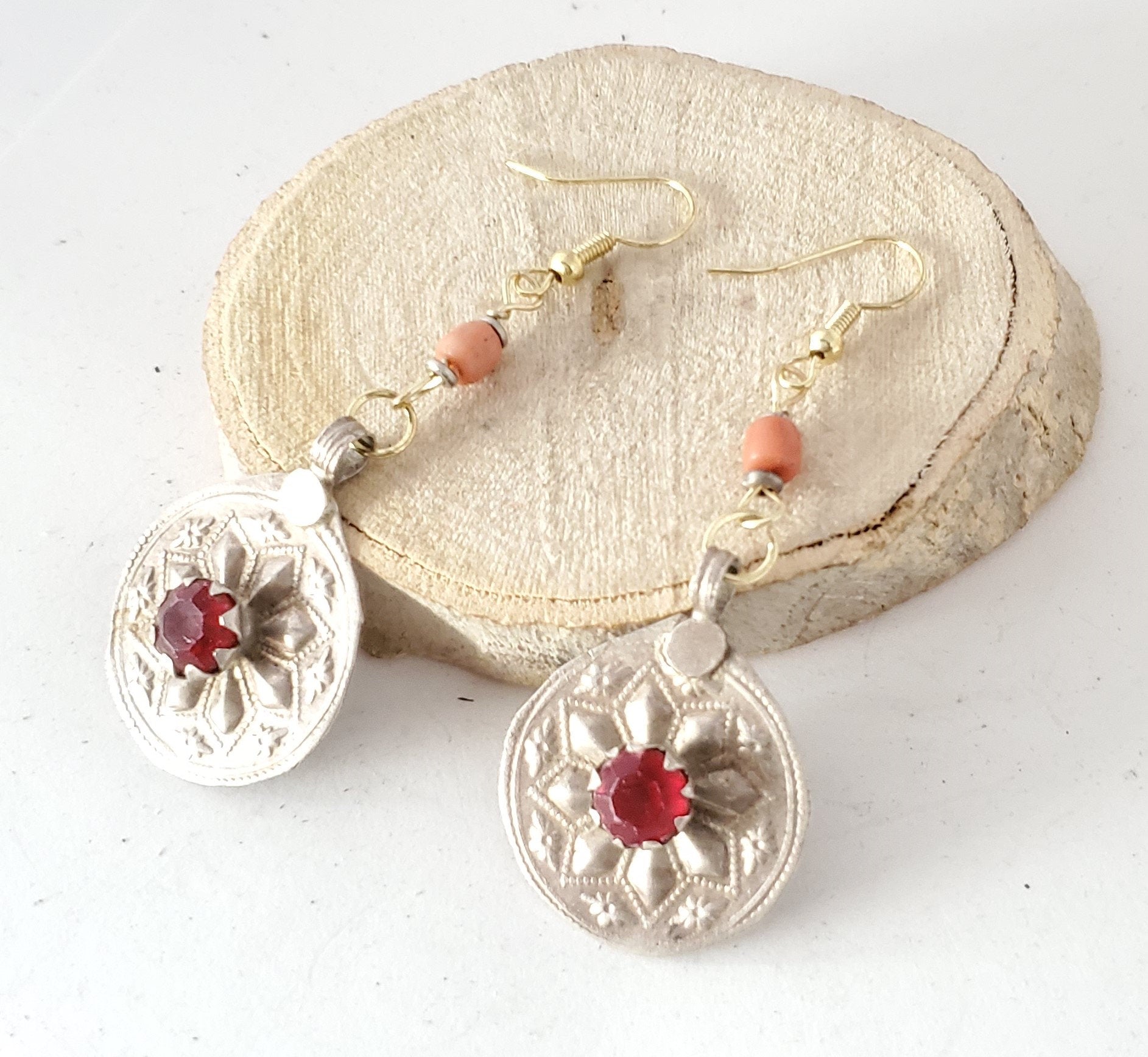This detailed color photograph showcases a pair of elegant dangle earrings designed for a product website. The earrings rest on a small, circular slice of light-colored wood, resembling a freshly cut tree branch, with bark clinging to its edges. The earrings feature gold hooks that attach to a series of beads: a coral bead sandwiched between two silver beads. Below the beads, a circular silver charm dangles, adorned with a stamped floral or star-shaped design, and a vivid red or maroon gem, possibly a garnet or ruby, at its center. The display is set against a plain white background, highlighting the earrings' detailed craftsmanship and the natural texture of the wood base. The composition includes a palette of delicate beige, metallic gold, silver, coral pink, and deep red hues.